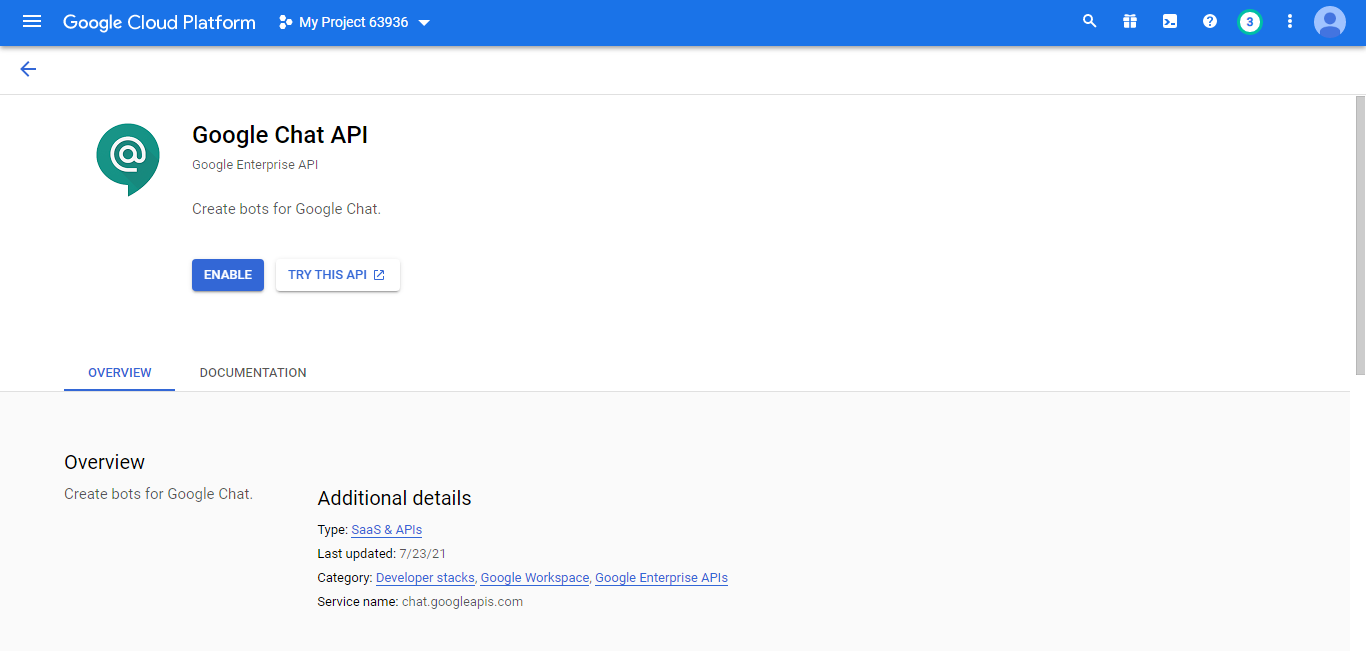The image depicts a screenshot of the Google Cloud Platform interface, showcasing the Google Chat API page. At the top, there's a full-width blue banner. On the upper left corner, a standard hamburger menu icon is displayed, accompanied by the text "Google Cloud Platform" in white. To its right, a "Projects" drop-down menu shows the project ID "63936," allowing users to select different projects. The upper right corner features typical browser icons, including a user profile icon and a search bar.

Below the banner, the main content area predominantly features a white background. An arrow on the upper left allows users to navigate back. Centered in this white space is a small green icon with the label "Google Chat API," followed by descriptive text. Below this description, there are two buttons: a prominent blue "Enable" button and a white "Try this API" button.

Further down, two tabs are visible: "Overview" and "Documentation." The "Overview" tab is currently selected, as indicated by the gray bar underneath it. The "Overview" section itself is divided into two columns of detailed information, including details on the API's type and the last update timestamps, with some clickable links for additional information.